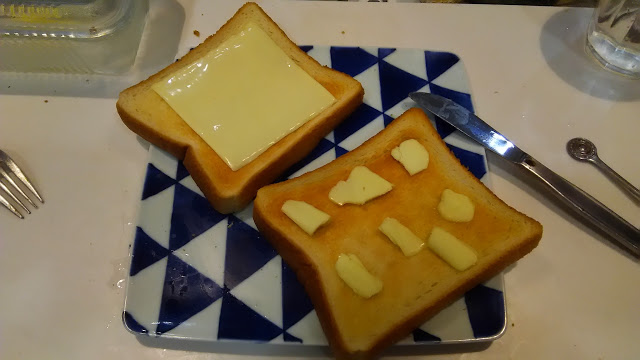This color photograph displays a white tabletop with a few crumbs scattered across its surface. Centered in the image is a square porcelain plate adorned with a repeating pattern of dark blue and white triangles forming a diamond-checked design. On the plate are two pieces of toasted bread. The piece at the top features a slice of pale yellow American cheese, while the piece at the bottom has several dabs of yellowish butter. The bread has a nicely toasted appearance, with the crust being a darker brown.

Flanking the plate on the left are the tines of a fork, positioned diagonally. To the right, a butter knife rests against the plate, and beside it lies a small, dark metal spoon. In the top left corner of the image, an indeterminate metallic object is visible, possibly a bowl. The top right corner reveals parts of a water glass, which casts a faint reflection on the white surface. The photograph captures a casual dining setup with a focus on the neatly presented toasted sandwich and accompanying utensils.